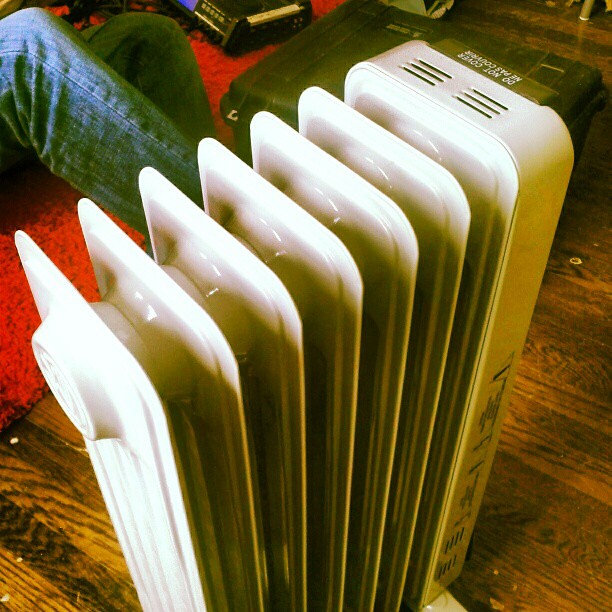The image, captured from a first-person perspective looking down in what appears to be someone's home or apartment, prominently features a white, portable electric radiator positioned centrally. This shiny metal radiator, which consists of multiple coils and vents, seems to be the focal point of the photograph. The background showcases a darker brown hardwood floor partially covered by a red shag rug. Additional details include a pair of bent legs clad in blue jeans, suggesting someone is sitting or kneeling near the radiator. Adjacent to the legs is a black object that resembles a toolbox or footstool. There's also an orange hue that adds a warm tone to the overall scene.